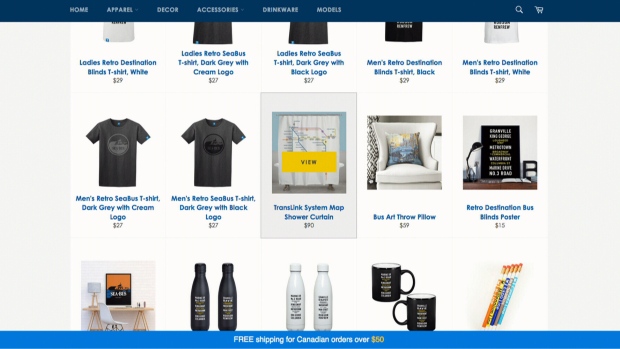Here is a clean and detailed caption for the described image:

---

This screenshot from a retail store website features a dark blue header at the top with navigation options for Home, Apparel, Decor, Accessories, Drinkware, and Models. To the right of the header, there is a search text box with a magnifying glass icon and a shopping cart icon.

The top row of merchandise includes:
- A Ladies Retro Destination Blinds T-shirt (white), priced at $21, now $29.
- A Ladies Retro C-Bus T-shirt (dark gray with a cream logo), priced at $27.
- A Ladies Retro C-Bus T-shirt (dark gray with a black logo), priced at $27.
- A Men's Retro Destination Blinds T-shirt (black), priced at $29.
- A Men's Retro Destination Blinds T-shirt (white), priced at $29.

In the middle row, we see:
- A Men's Retro C-Bus T-shirt (dark gray with a cream logo), priced at $27.
- Another Men's Retro C-Bus T-shirt (dark gray with a black logo), priced at $27.
- A clickable image of a shower curtain with a map on it, labeled "TransLink System Map Shower Curtain," priced at $90.
- A white chair with a throw pillow labeled "Bus Art Throw Pillow," priced at $59.
- A sign with white letters on a black background, noted as a "Retro Destination Bus Blinds Poster."

The bottom row includes images of the following items, but without visible text descriptions:
- A table with a blue and orange poster above it.
- A pack of two black water bottles.
- A pack of two white water bottles.
- A set of two black mugs.
- Five pencils, each in a different color.

At the bottom of the screen, a blue footer states, "Free shipping for Canadian orders over $50."